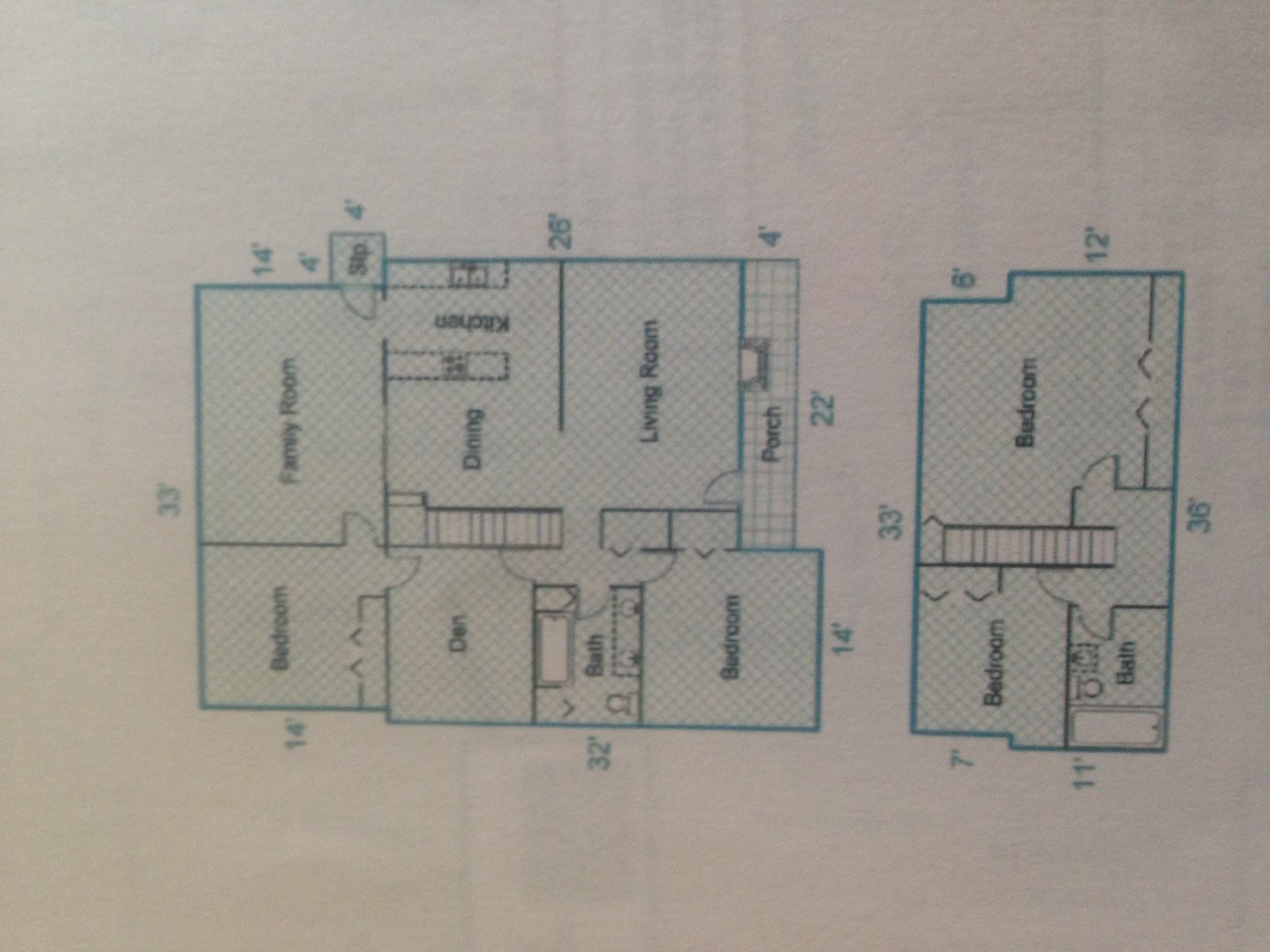The image displays a rudimentary, hand-drawn blueprint of a residential property, possibly a house or a condo. The blueprint appears to be oriented on its side. Starting from the left, the labeled rooms include a bedroom, followed by a family room, a den, and a dining area. Then, there is a living room, another bedroom, and yet another bedroom. On what seems to be the second floor, the blueprint shows additional bedrooms and a bathroom. Each room is annotated with various measurements, some of which include 33, 14, 32, 26, and 4, indicating the dimensions of each corresponding space.